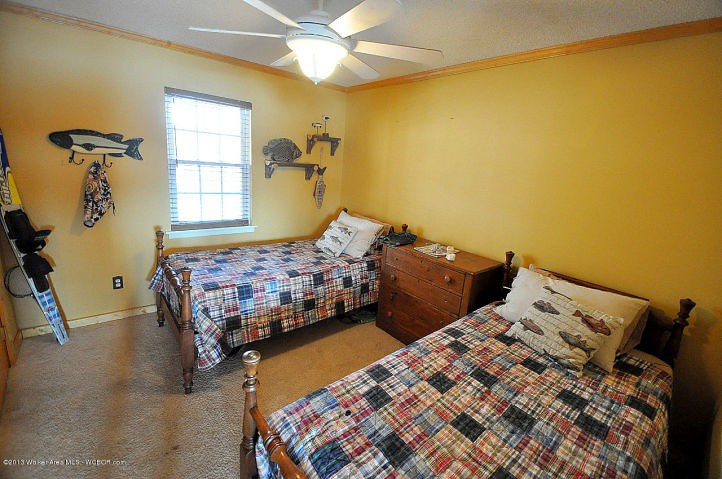This high-quality image depicts a brightly lit bedroom, seemingly staged for a hotel advertisement or an Airbnb listing. The room features two twin beds aligned at an angle, each adorned with multi-colored checkered quilts and matching pillows, one off-white and the other showcasing a fish design. The beds have classic headboards and footboards and are separated by a wooden chest of drawers with four spacious drawers, serving as a functional centerpiece. The walls of the room are painted a cheerful yellow and decorated with various items, including a mounted wooden fish used as a hook to hang bags. Additional wall accents include shelves displaying knick-knacks and a single slalom water ski propped against the wall on the left. The floor is covered in brown carpeting, adding a warm and cozy feel to the space. A window with blinds allows natural light to stream in, further illuminating the room, and a six-bladed ceiling fan is positioned at the center of the ceiling. The combined elements create a welcoming and well-coordinated interior.